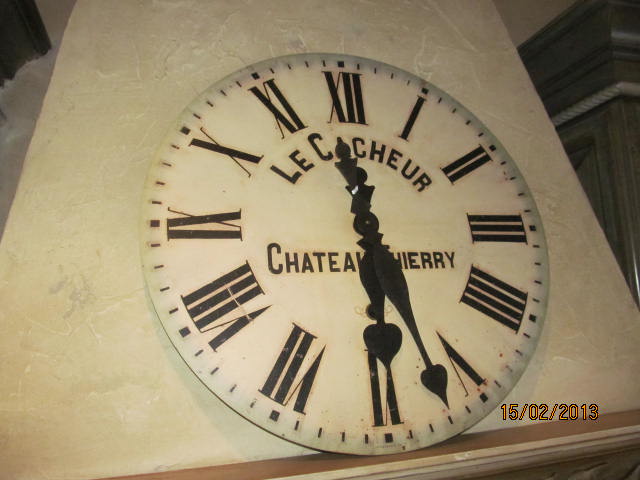In this image, we have a detailed view of a crafted stone piece featuring an integrated clock. The stone, adorned in hues of white, silver, and cream, exhibits meticulous craftsmanship. The clock is seamlessly set into the stonework, resting just above a ledge-like shelf which may be constructed of either wood or a matching stone material. To the right side of the image, there is a timestamp reading "15/02/2013" in orange. The clock, harmonizing with the stone's aesthetics, bears an inscription, though partially obscured, reading "LE SEE C HE...CHA E A TE I E R R...". The clock's hands indicate the time as 6:37.